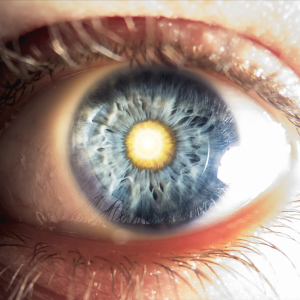This is an extremely close-up photograph of a human eye, showcasing remarkable detail. The skin around the eye is pink, with light brown eyelashes framing the scene. The sclera (white part of the eye) contrasts strikingly with the multifaceted iris, which is predominantly blue but interspersed with various shades of blue and gray, creating a cloudy, streaky pattern with small gaps or holes. The most captivating feature is the pupil, which dramatically deviates from the norm by being a bright, glowing yellow, resembling a small sun. This unusual coloration could be a reflection from an external light source, suggested by the glare visible on the eye’s surface. The meticulous detail hints at professional photography, although it might also be the result of an amateur using a high-quality camera. The image is rich with colors including black, white, gray, yellow, blue, pink, brown, and possibly some red, but it focuses solely on the eye without any additional context or surrounding features such as the eyebrow.